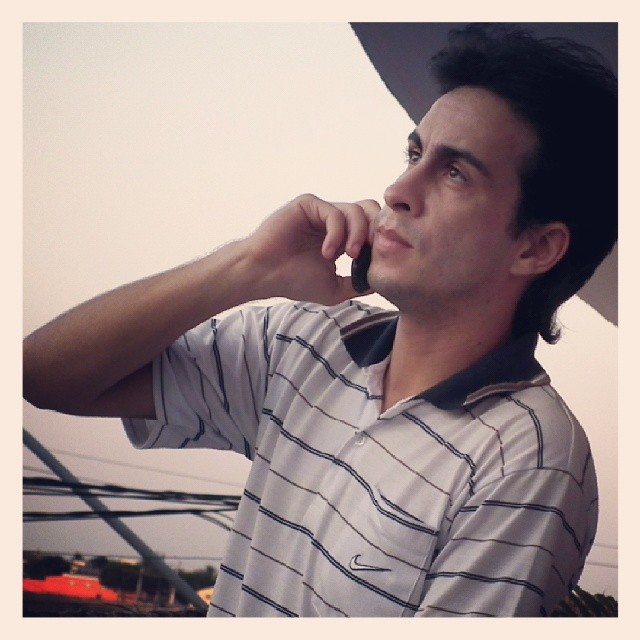This photograph depicts a Caucasian man engaged in a phone conversation, holding a small, retro flip phone in his right hand. The man's attire is characteristic of the late 90s to early 2000s, featuring a white polo shirt with blue stripes and a Nike swoosh, accentuated by a blue collar that is somewhat open. His dark hair is styled with a swoop over and back, giving him a stern expression as he looks towards the left corner of the image. The scene takes place outdoors, during what seems to be a hazy, possibly sunset moment. In the background, the setting includes telephone wires, power lines, and buildings, along with a visible canopy or roof in dark gray above him. There's a red building with a beige roof and trees far off into the distance, contributing to the overall atmosphere. A light pink border frames the image, and elements like the pole and wires create a dynamic composition within the scene.